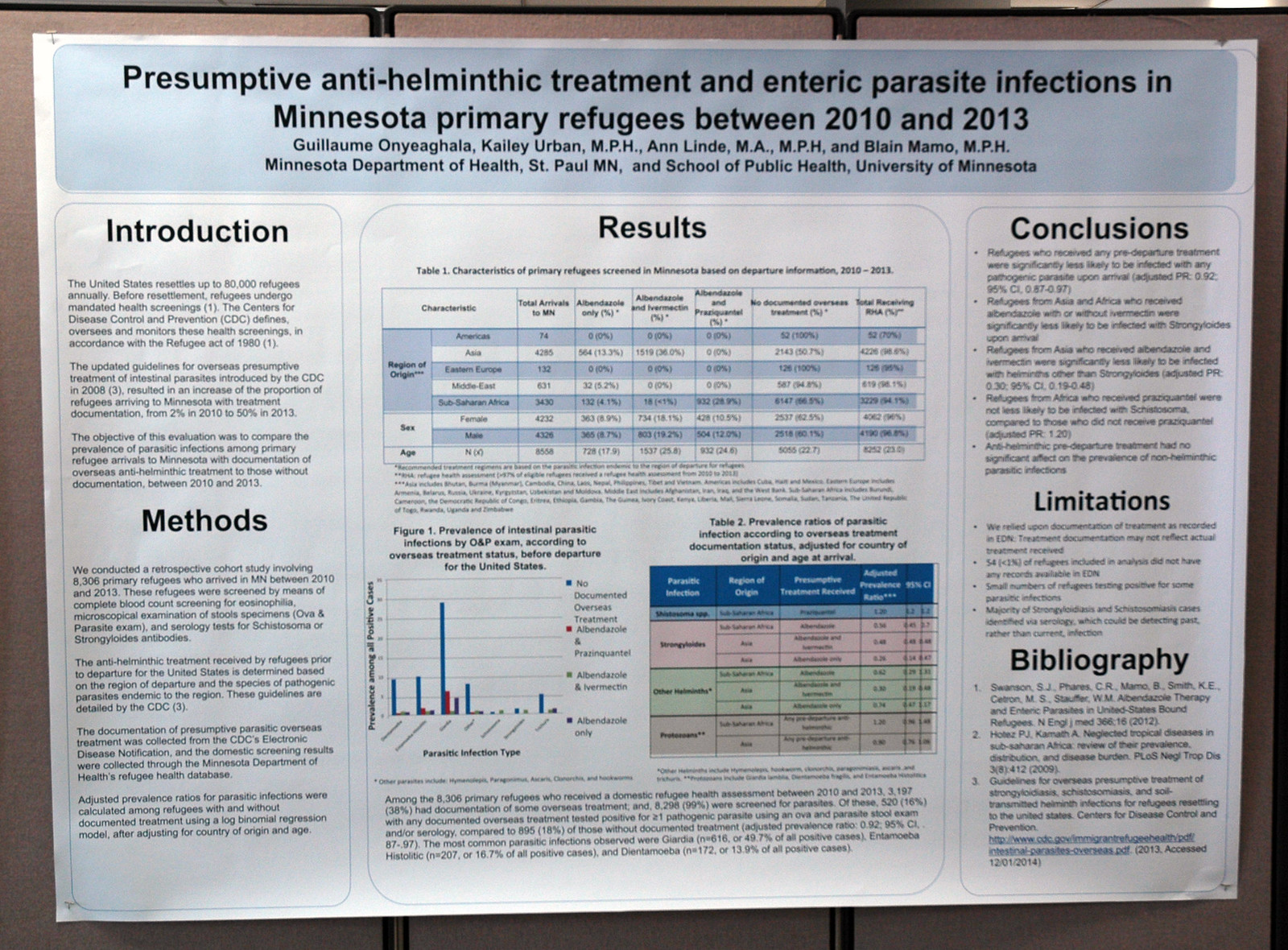The image depicts a conference poster titled "Presumptive Anti-Helminthic Treatment and Enteric Parasite Infections in Minnesota Primary Refugees between 2010 and 2013" displayed on a beige background. The title is prominently featured at the top on a blue banner. The poster is sectioned into three vertical columns. 

On the left column, which takes up about one-quarter of the poster, there are sections titled "Introduction" and "Methods," each with accompanying text in black on a white background. 

The central column, occupying approximately half of the poster's width, is dedicated to "Results." This section includes a grid-style data chart and a bar graph on the lower left side, as well as a colored chart with parts in pink, blue, and gray on the right.

The right column, also taking up about one-quarter of the space, features "Conclusions" with a bulleted list, "Limitations" with another bulleted list, and a "Bibliography" citing three sources. Several authors' names are listed beneath the title, including a prominently difficult-to-pronounce name spelled G-U-I-L-L-A-U-M-E O-N-Y-E-A-G-H-A-L-A. The poster is arranged in a manner typical for scientific conference presentations, designed for summarizing the study’s introduction, methods, results, conclusions, limitations, and references.